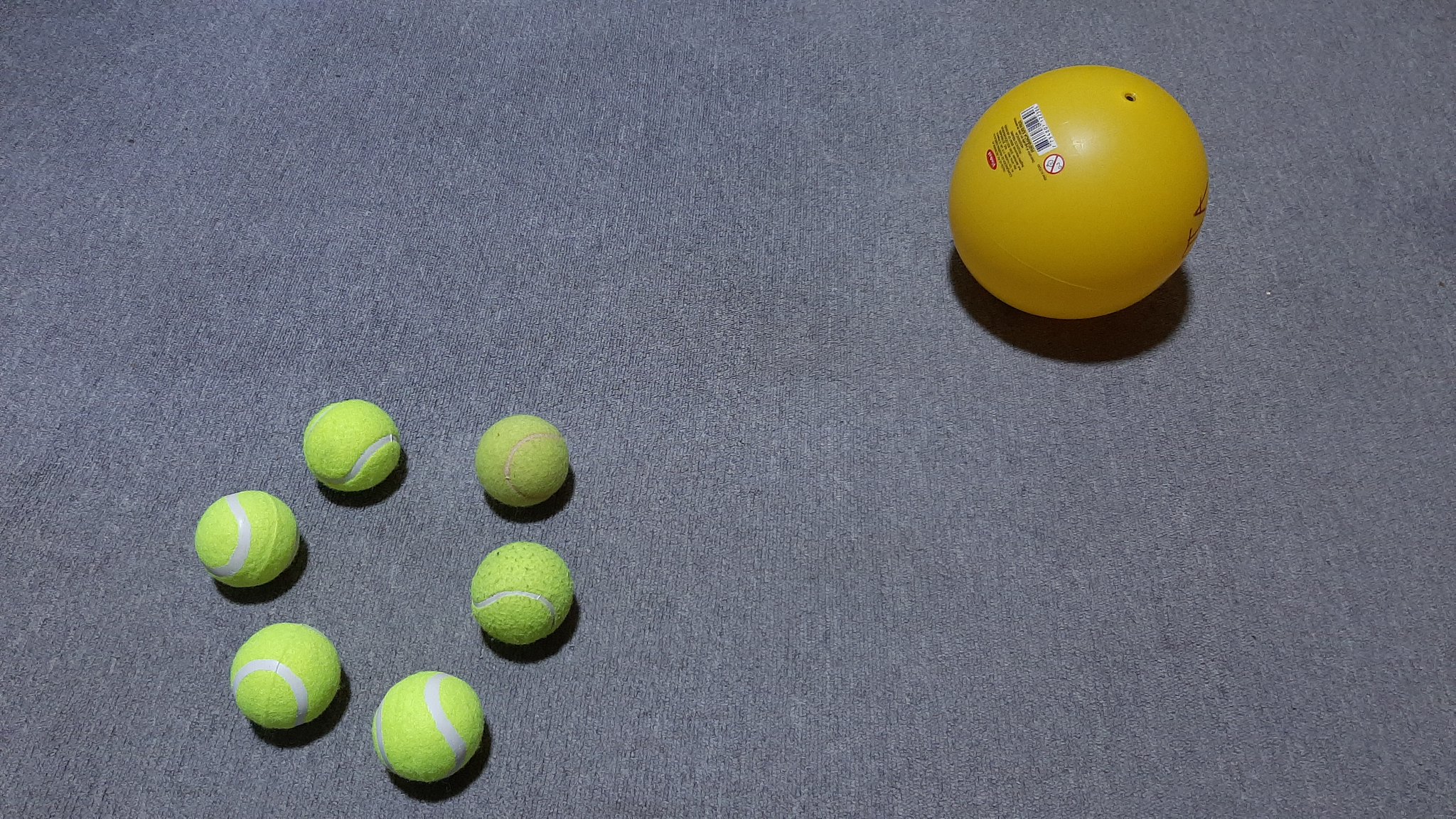This image, taken from an overhead perspective, displays two types of balls resting on a textured gray carpet. Positioned near the bottom left, six tennis balls form a circular pattern with an empty center. These tennis balls vary in their condition, ranging from bright lime-colored and new to progressively dirtier, indicating varying levels of use. Notably, the tennis ball closest to the other ball is the dirtiest among them. To the top right, a single yellow dodgeball stands out. This dodgeball, filled with air, features a visible white barcode label with small black print above it, and an inflation section marked as a small black dot. The yellow ball casts a darker, orangish shadow with a more intense shadow area beneath it, adding depth to the image.